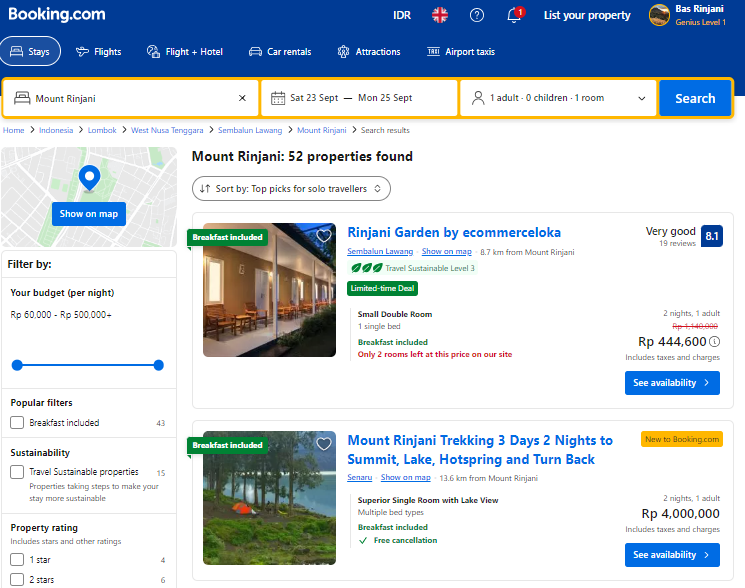**Detailed Caption:**

This image is a detailed screenshot of the Booking.com web page interface. In the upper left-hand corner, the Booking.com logo is prominently displayed. On the upper right-hand corner, a user's profile information is visible. The user's name appears to be *BaRinjani*. Beneath the name, the account status is indicated as *Genius Level 1*, accompanied by an icon featuring a nature photograph on the left side. To the left of this section, there is an option labeled *List your property*.

Further to the left, four icons are neatly arranged: the first represents the currency IDR, the second features a plus sign with a sunburst, the third is a question mark within a circle, and the fourth is a bell showing one alert notification.

Directly beneath this row, the navigation menu displays six main categories: *Stays*, *Flights*, *Flight + Hotel*, *Car Rentals*, *Attractions*, and *Airport Taxis*. The *Stays* category is highlighted, and the search bar is active, showing the destination *Mount Rinjani*. The calendar is set from Saturday, September 23, to Monday, September 25, for one adult with zero children in one room.

Below, a breadcrumb navigation trail reads: *Home > Indonesia > Lombok > West Nusa Tenggara > Mount Rinjani*. The main section shows search results with the heading: *Mount Rinjani: 52 properties found*.

The first listing features a prominent image of a hotel front with tan-colored walls, white porch bases, pillars, and greenery. To the right, the listing details are provided: *Rinjani Garden by e-commerce Loka*, rated 8.1/10 from 19 reviews in blue text. It further notes the location as 8.7 kilometers from Mount Rinjani and boasts *Travel Sustainability Level 3*. This listing highlights a *Limited time deal* for a *Small double room with one single bed, breakfast included*. Only two rooms are available at the displayed price of RP 444,600 for two nights, for one adult, including taxes and charges. Users are prompted to check availability for booking.

The second listing showcases a campsite image with trees, a lake, and green grass. The description mentions a *Mount Rinjani Trekking: 3 days, 2 nights to summit, lake, hot spring, and return*. Financial details note a price of RP 4,000,000 for this experience.

On the left side of both listings, filters are available to refine search results by budget (RP 60,000 to 500,000), breakfast included, and other customizable options.